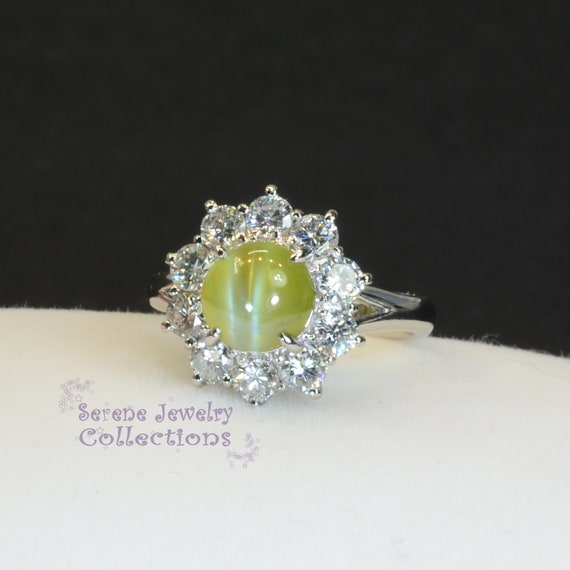This image features a highly detailed, color photograph of a silver ring from the Serene Jewelry Collections. The ring showcases a central, iridescent greenish-yellow stone, with striking variations such as blue lines, bubbles, and white spots. Surrounding the central gem is a halo of large, clear diamonds arranged in a floral pattern. The diamonds are held securely by prongs, emphasizing their size and clarity. The ring is positioned on a white surface, possibly fabric or a cushion, against a black background. Beneath the ring, the text "Serene Jewelry Collections" is visible in purple, adding a luxurious and branded element to the overall presentation. The combination of the sparkling diamonds and intricate details of the central stone make the ring exceptionally shiny and visually captivating.